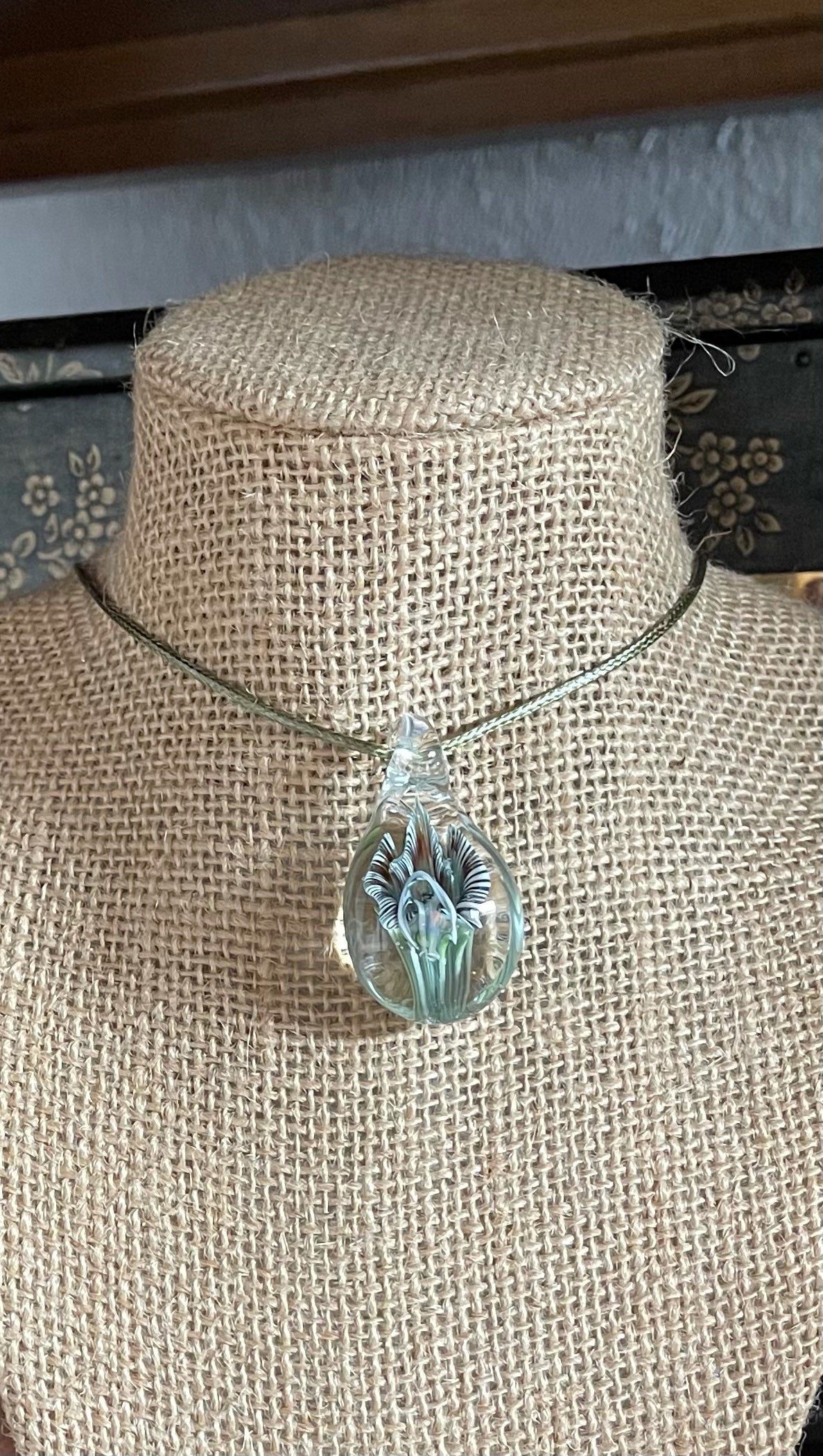The photograph captures a headless, armless mannequin covered in a burlap-like material, sitting on what appears to be a chest. The mannequin features a choker-style silver chain, or silver rope, adorned with a beautiful clear pendant. This pendant contains intricate details that seem to depict a person alongside delicate elements reminiscent of flowers or leaves, hinting at shades of blue and light green. In the background, a white wall complements the scene with possible floral accents, suggesting an artistic or store display. The overall composition hints at elegance and beauty, with the necklace glimmering under light, likely as part of an advertisement for a fine jewelry store.